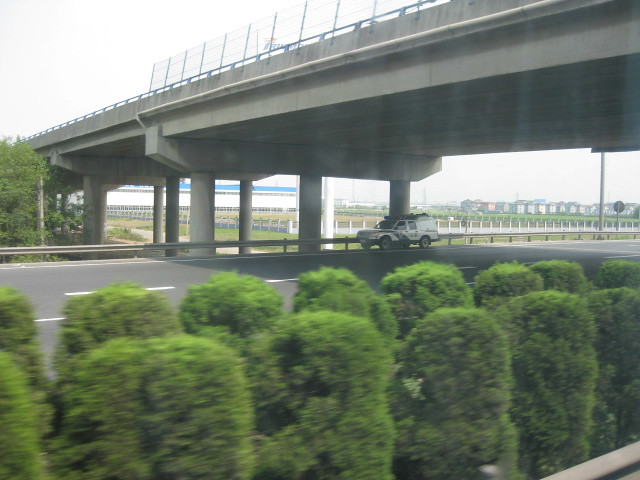The photo depicts a slightly blurred scene featuring a highway with a prominent overpass overhead. A white truck with a distinct blue stripe running along its side and front, accompanied by an indistinct blue object on its roof, appears to be parked beneath the overpass. The asphalt of the highway looks clean and fresh, highlighted by guardrails that provide safety barriers both on the road and on the overpass. The vantage point of the photo seems to be from behind several green bushes that appear slightly blurred, potentially due to the motion of the photographer. 

In the distance, a large white building with a blue roof is visible, which might be a factory or warehouse, alongside numerous power poles. To the right, there are smaller buildings that could be apartments, although they are too far to definitively identify. The sky above is a muted whitish-gray, adding a calm yet overcast feel to the composition. The overall landscape, architecture, and the type of vehicle suggest that the location might not be in the United States, with possibilities of it being in Europe or Japan.